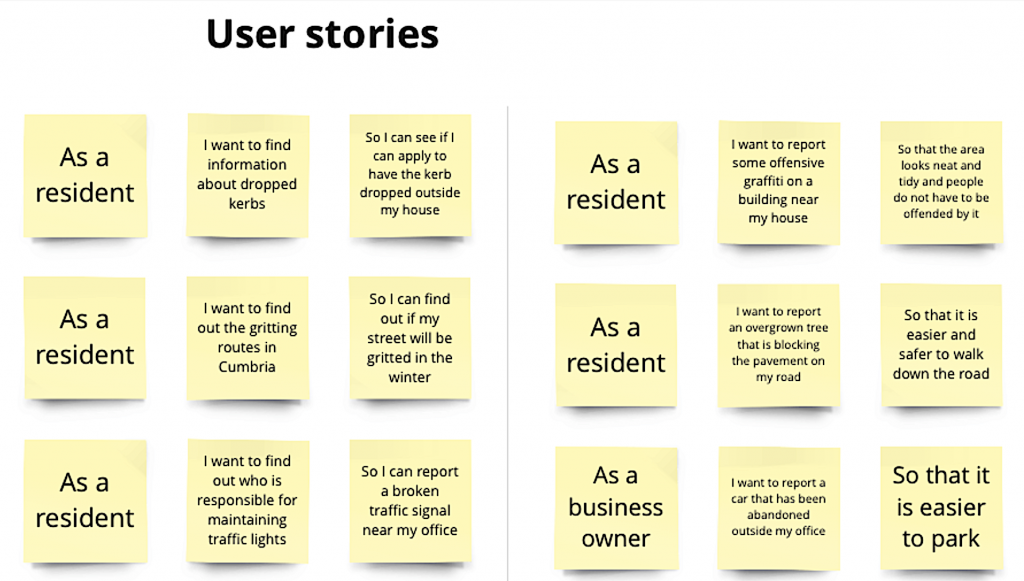The image is a digital rendering of a chart composed of 18 light green, sticky note-style squares, arranged in two vertical grids of nine notes each, separated by a thin gray line. The background is white. At the very top left corner of the image, the title "User Stories" appears in large black sans-serif font. Each sticky note on the left column of both grids prominently features the phrase "As a resident" in the same black sans-serif font. The notes detail various concerns residents have, including a desire to find information about applying for dropped curbs outside their homes, reporting offensive graffiti to ensure neighborhood tidiness, inquiring about gritting routes in Cumbria during winter, reporting overgrown trees obstructing pavements, and determining who is responsible for maintaining traffic lights to report a broken signal near an office. Each sticky note casts a small shadow, adding depth to the digital rendering.